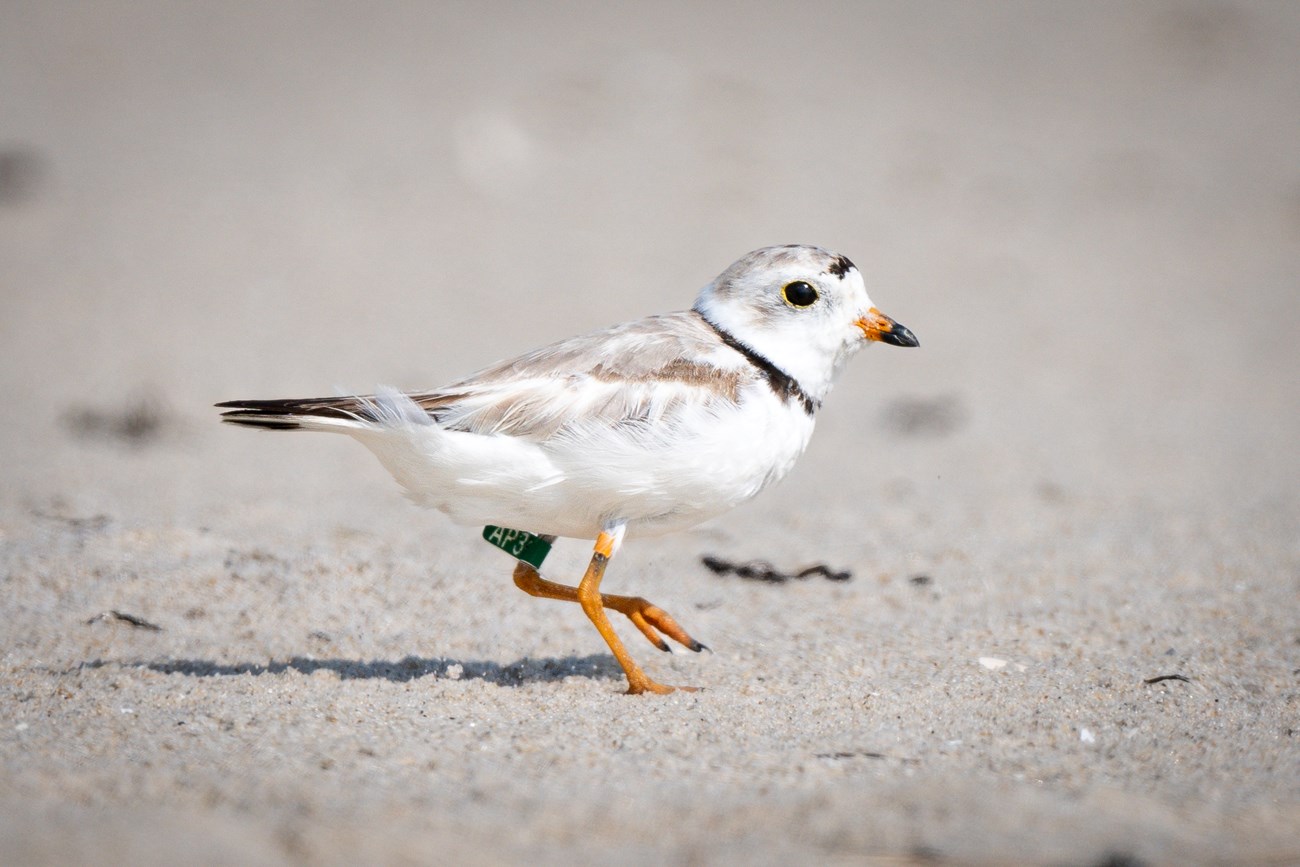This is a detailed close-up photograph of a small, white bird that appears to be a sandpiper. The bird is predominantly white but has a range of other colors accentuating its features. Its beak is orange with a distinctive black tip. The bird's eyes are beady and black. Dark spots and flecks can be seen on the top of its head, around its eyes, neck, and back, adding to its detailed plumage. Additionally, light brown flecks adorn its feathers, notably around its back, neck, and tail, which has darker brown feathers. The bird is standing on one leg on what looks like a beach, with fine grains of beige sand beneath it. Its legs are orange, and attached to its left leg is a thin green tag labeled "AP3" in small white letters, suggesting it might be part of an experiment or study. The overall scene highlights the bird's delicate and intricate features, set against the soft, sandy background of a beach.